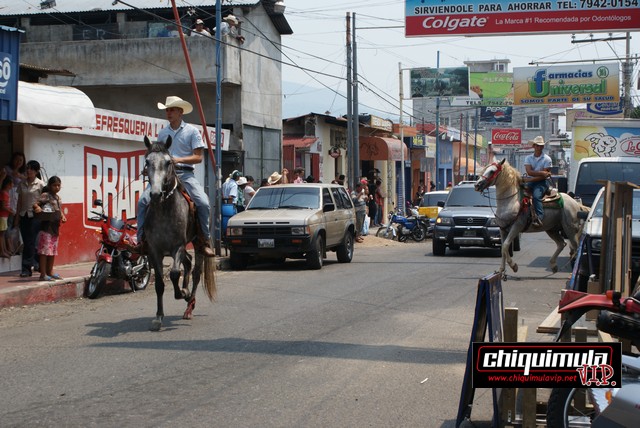In a bustling street that appears to be in either Puerto Rico or Mexico, two men are seen riding horses down the middle of a paved road. The men, dressed similarly in white cowboy hats, light blue polo shirts, and jeans, exude a vibrant and confident presence. The tan and brown horses they ride further add to the picturesque scene. Surrounding them are older buildings adorned with aged awnings, bearing signs such as "Frescaria." Street poles are lined with colorful banners in hues of green, light green, orange, and red, with a prominent Colgate banner in red and white prominently displayed overhead. The street is lively, with SUVs driving slowly and parked cars, indicating a busy town or village atmosphere. Pedestrians line the sidewalks, engrossed in watching the horse riders pass by, creating an engaging and dynamic daytime snapshot of the local culture.